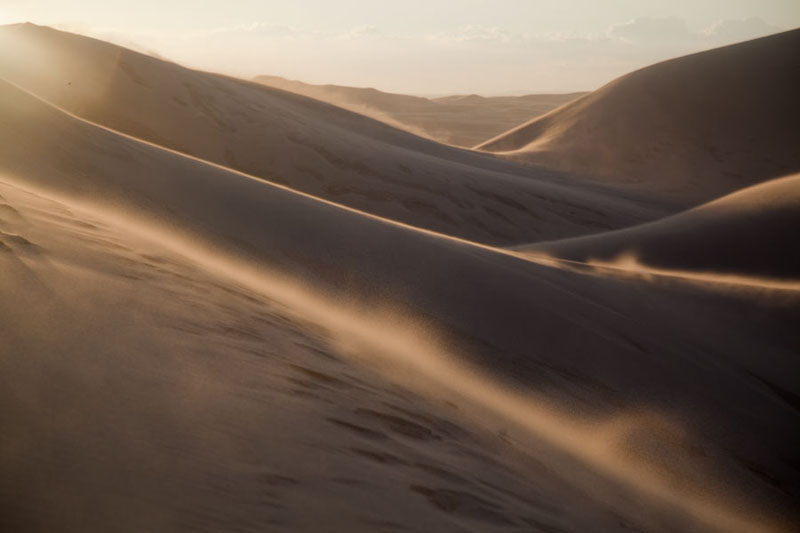A mesmerizing photograph captures the grandeur of a desert landscape at sunrise or sunset, revealing an expanse of towering sand dunes bathed in a reddish-brown hue. The foreground is dominated by a large dune that diagonally spans the left third of the image, its outline softened by the wind stirring up a fine layer of dust. Visible footprints trail across this dune, adding a human touch to the vast, undulating terrain. In the top left corner, the sun casts a radiant glow, creating deep, almost black shadows that carve out the dunes' intricate shapes and contours. The areas where the sunlight touches the sand are illuminated in a strikingly bright caramel color, providing a breathtaking contrast. The sky above is awash with a honey gold yellow, punctuated by wisps of clouds. The scene is further enriched by the presence of numerous dips and valleys, with dunes rising and falling rhythmically across the landscape, showcasing the desert's dynamic and ever-changing topography.